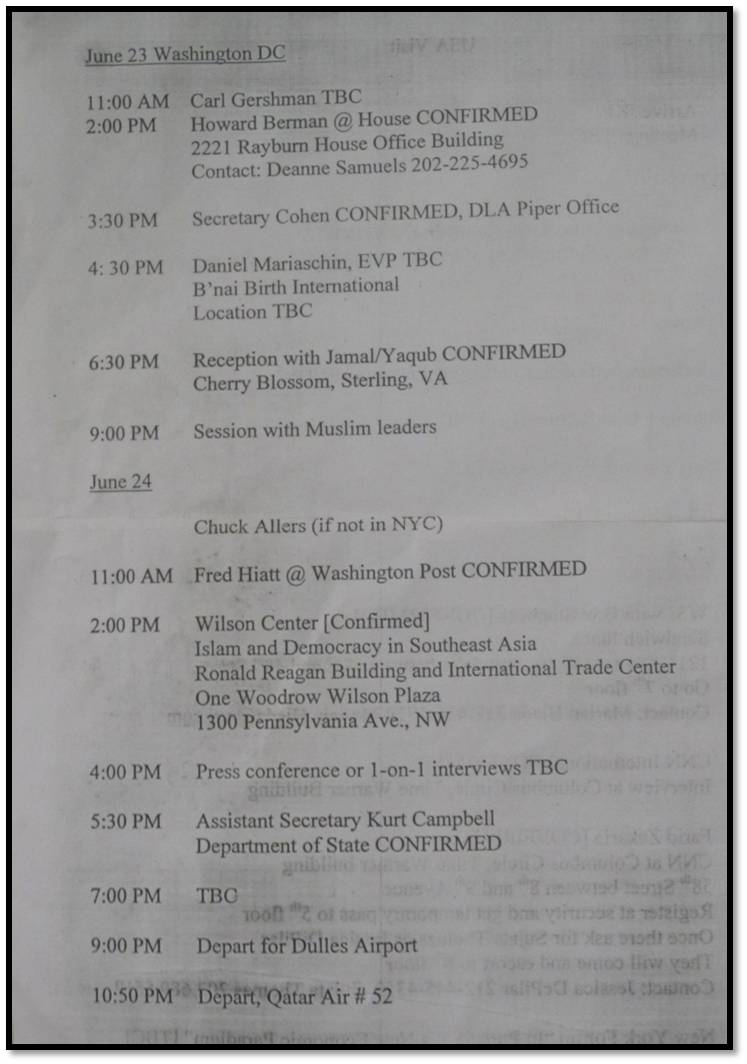**Detailed Agenda of Events for June 23rd and 24th:**

**June 23rd – Washington, D.C.:**
- **11:00 AM:** Call with Geersman (To Be Confirmed)
- **2:00 PM:** Meeting with Howard Berman at his house (Confirmed)  
  *Location:* 2211 Rayburn House Office Building  
  *Contact:* D.N. Samuels (202-225-4695)
- **3:30 PM:** Meeting with Secretary Cohen (Confirmed)  
  *Location:* DLA Piper office
- **4:30 PM:** Meeting with Danielle Maria Shin, EVP (To Be Confirmed)  
  *Location:* B'nai B'rith International (Location To Be Confirmed)
- **6:30 PM:** Reception with Jamal Jacob (Confirmed)  
  *Location:* Cherry Blossom, Sterling, VA
- **9:00 PM:** Session with Muslim Leaders

**June 24th – Washington, D.C.:**
- **11:00 AM:** Meeting with Fred Hyatt at The Washington Post (Confirmed)
- **2:00 PM:** Event at Wilson Center (Confirmed)  
  *Topic:* Islam and Democracy in Southeast Asia  
  *Location:* Ronald Reagan Building and International Trade Center, 1 Woodrow Wilson Plaza, 1300 Pennsylvania Avenue NW
- **4:00 PM:** Press Conference or One-on-One Interviews (To Be Confirmed)
- **5:30 PM:** Meeting with Assistant Secretary Kurt Campbell at the Department of State (Confirmed)
- **7:00 PM:** Slot To Be Confirmed
- **9:00 PM:** Departure for Jules Airport
- **10:50 PM:** Depart via Qatar Air No. 52